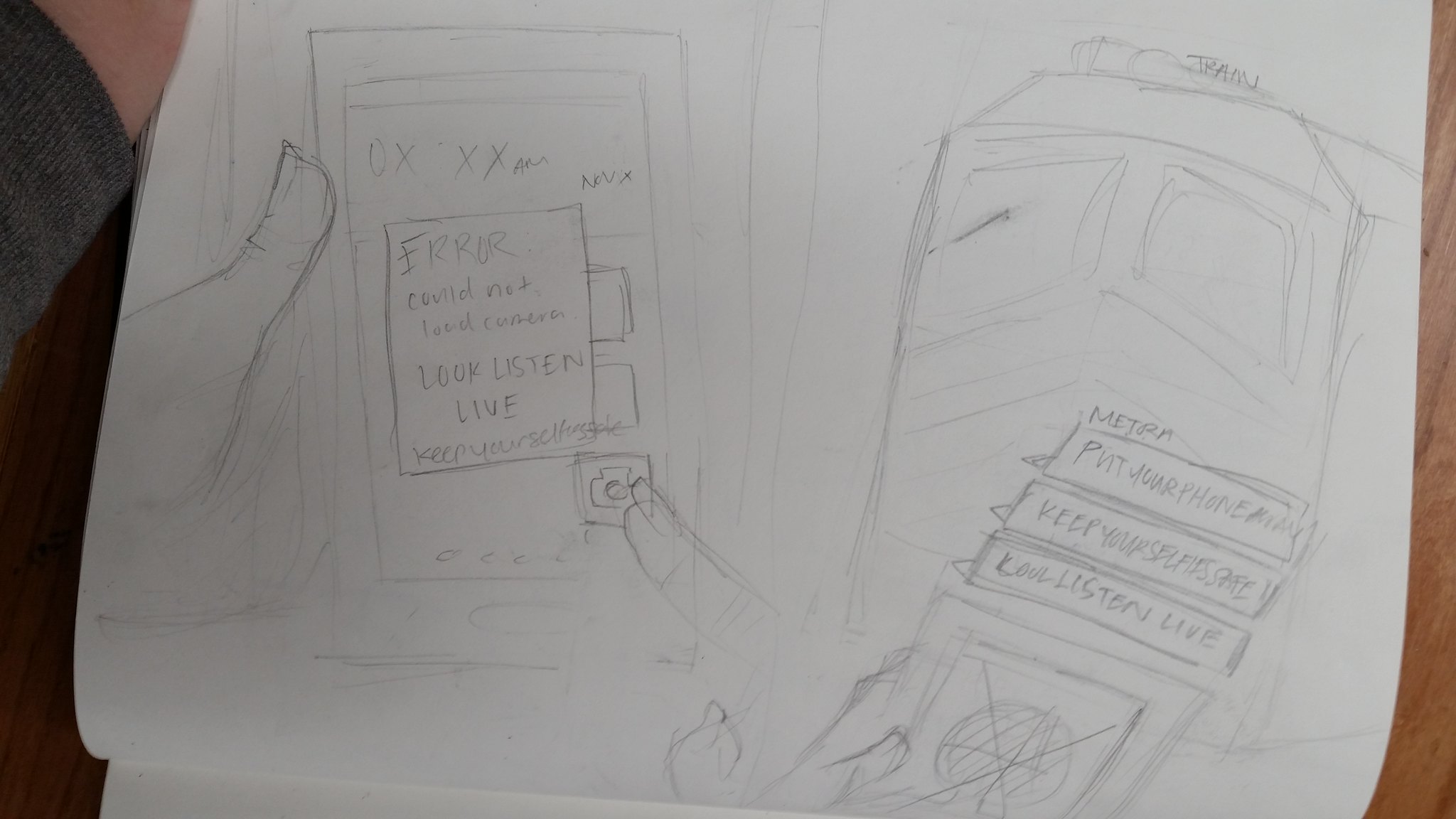This highly detailed pencil drawing is on a white sheet of paper, laid on a wooden surface. The main focus of the drawing is a hand holding a large, square tablet device, capturing the intricate detailing of each finger and thumb. The other hand of the person is depicted as pressing a button on the tablet. At the top of the tablet screen, the text "OXXX" is visible. The screen also displays a square area intended to represent a picture or digital content, labeled "COVID test or something," followed by "100 listen live." Additional tabs extend from this main section. To the right of the tablet screen, there appears to be a secondary image within the drawing, showcasing a person holding a clipboard containing sketches and text at its top. Above this, there is a depiction of what seems to be the front of a train, adding a further layer of complexity and narrative depth to the artwork.